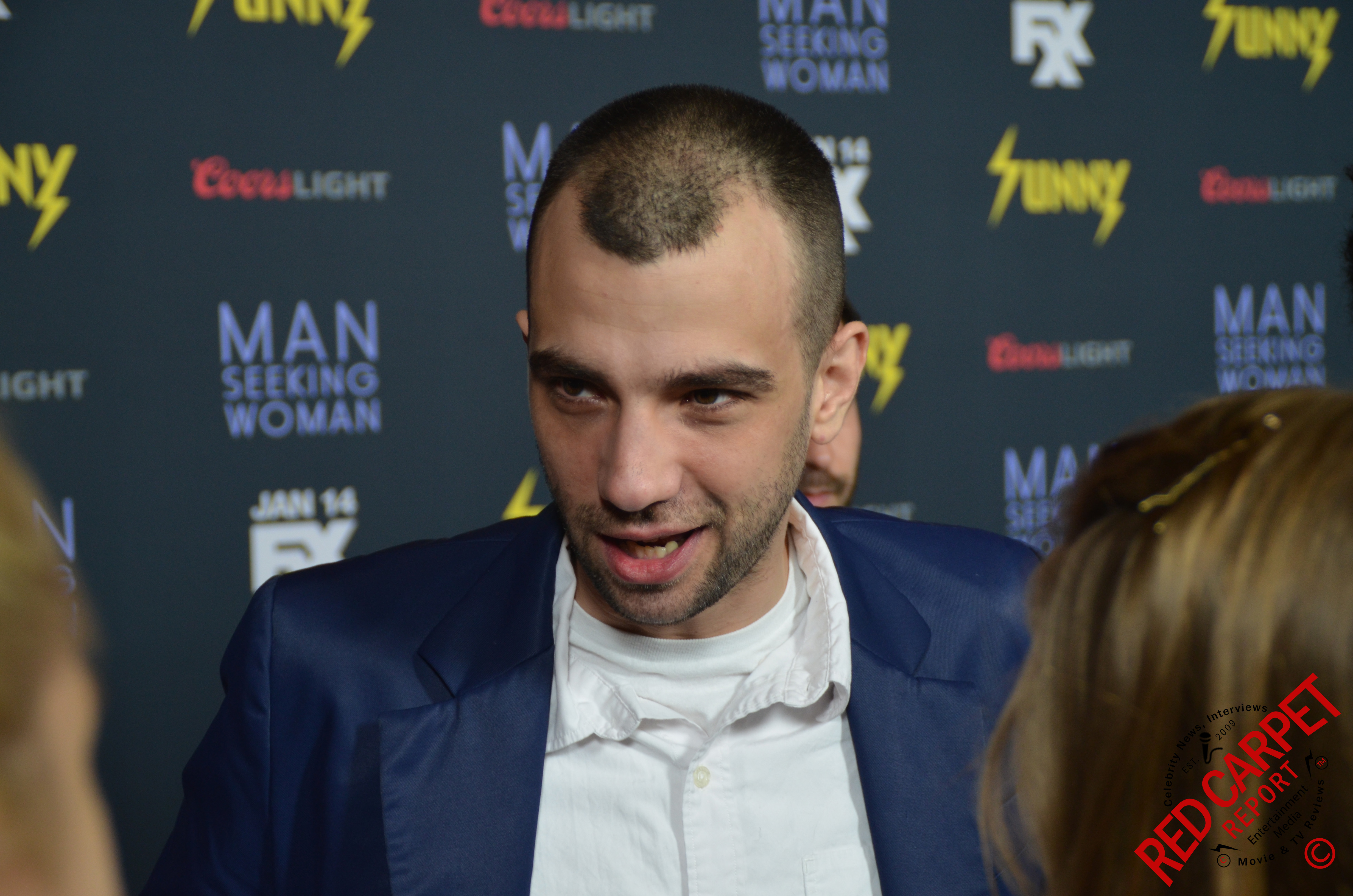In the image, a man in the center of the photograph is at a red carpet event, wearing a blue blazer over a white button-up shirt with an unbuttoned collar, revealing a white undershirt. He has very short hair, a noticeable five o'clock shadow, and appears to be looking slightly down to his left, possibly speaking to someone just out of the frame whose hair or face tips are faintly visible. The background features a dark gray or black wall adorned with various company logos, including "Coors Light" in red cursive text, "Man Seeking Woman" in blue, and "January 14 FX" in white. Additionally, a logo for "Sunny" in stylized yellow print appears multiple times along with numerous other indistinct logos. The setting suggests an indoor environment, characteristic of a red carpet event. The image is visually enhanced with a mix of colors including dark blue, yellow, red, gray, light blue, brown, and tan.